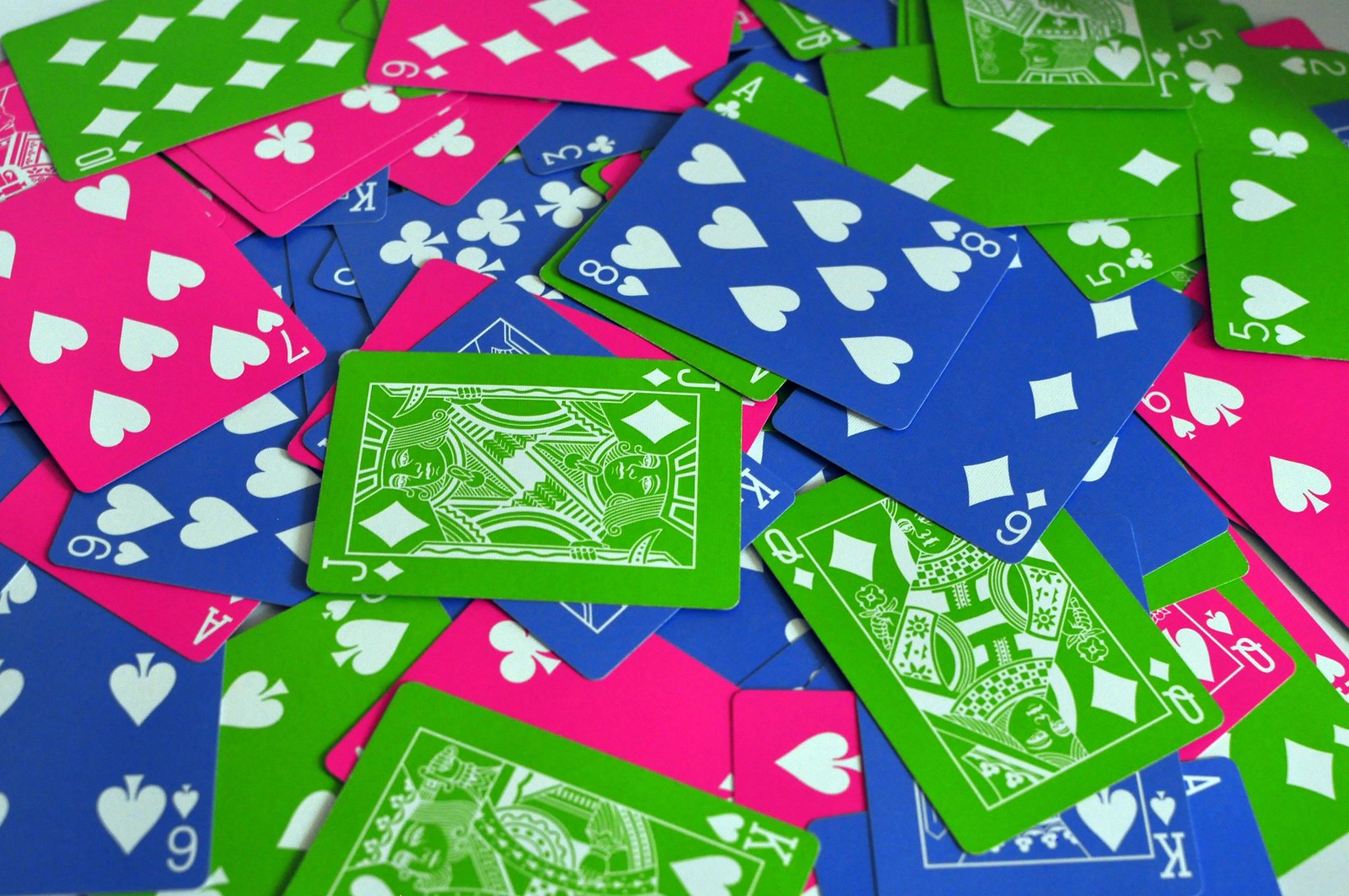A vibrant array of playing cards is sprawled across the table, showcasing a kaleidoscope of colors including bright green, dark blue, and hot pink. In the top left corner, a green 10 of Diamonds is partially covering a hot pink 7 of Hearts. Nearby, a hot pink 9 of Diamonds adds to the colorful display. Centrally located is a green Jack of Diamonds amidst an 8 of Hearts in dark blue, a green 5 of Hearts, a green 5 of Clubs, and a green 2 of Hearts at the top right. The bottom right features a dark green 8 of Diamonds alongside a dark blue 6 of Diamonds and a hot pink 5 of Spades positioned in the middle right. Further on the bottom right, a hot pink 8 of Spades and a King of Spades draw attention. On the bottom left, there's a King of Hearts, a 6 of Spades, and a 9 of Hearts. Completing the arrangement is another Jack of Diamonds in the middle left.